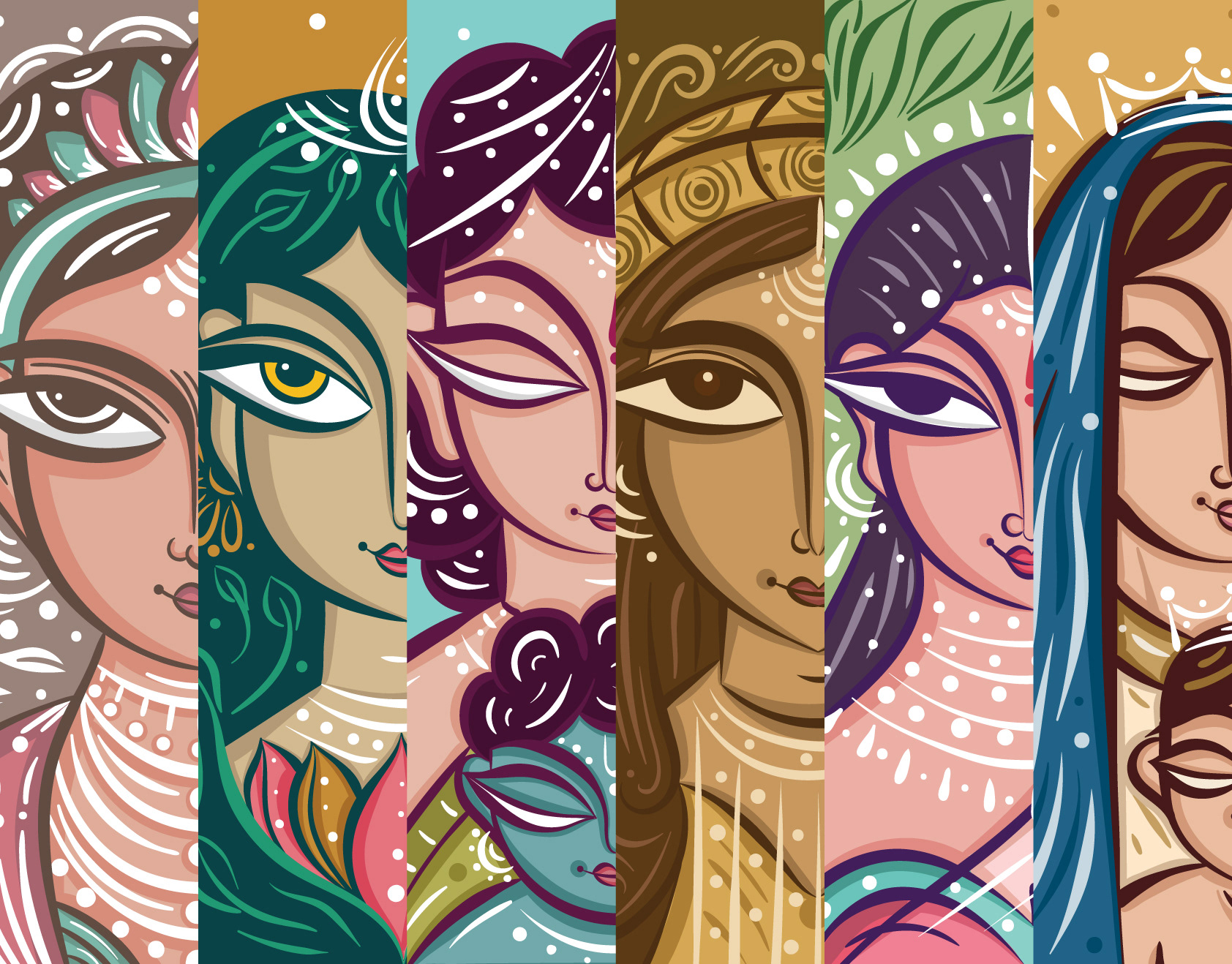The illustration is a vibrant cartoon artwork, featuring a collage of six horizontal panes, each depicting the right side of an Indian woman's face and neck in traditional attire. Each pane showcases half of the woman's face, from the top of her head down to her chest, capturing different shades and colors.

The detailed compositions show various color palettes, including yellows, greens, pinks, blues, and browns. The woman has dark hair across all panes, styled differently - in some, adorned with a tiara or jewelry, and in others, covered with a cloth. Her skin tone varies from red to darker shades, and she sports pink lipstick in several panes. Notably, the only visible feature of her face in every pane is her right eye, which is alternately open or closed. Her expressions are subtly intricate, with a consistent gentle smile.

The backgrounds and other elements also shift between panes. One pane features a blue background with the woman’s dark purple hair beside it; another depicts a green background against her pink skin and dark hair. In some panes, she appears alone, while in others, a child with similar brown hair is partially visible beside her. Her eyes differ in their details as well - some being yellow, others brown.

Intriguingly, the artwork also includes what looks like tattoos on her neck, enhancing the traditional aesthetic. Emphasizing a mix of cultural richness and individual beauty, the collage captures the essence of traditional Indian women through varied yet harmonious portrayals.